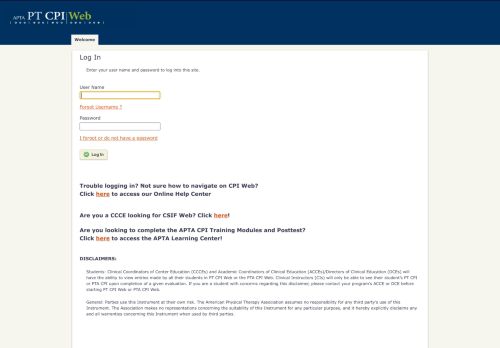A low-resolution screenshot of the PTCPiWeb website is displayed, showing an indistinct view of its elements due to poor image quality. At the top left corner, obscured but partially readable, is the company name "PTCPiWeb." Below the company name, there is a single tab labeled "Welcome," next to a "Log In" option, indicating that this is the login page of the website.

The central portion of the page instructs users to enter their name and username to log in. From the faint text, it appears to say "Login to the site". Below this, there is a text field labeled "Username" with a sample user name, such as "Avana", entered. An option labeled "Forgot Username" is positioned below the username field.

Further down, there is a password entry field, accompanied by a "Forgot Password" link, suggesting users can reset their password via email. Immediately below this, there is a gray login button featuring a green checkmark.

Towards the bottom of the page, under "Trouble Logging In," the text advises users to click a link for access to the online help center if they are having difficulties. Additional sections address specific users: one prompt asks if they are a CCCE looking for CSIF Web, while another inquires if they need to complete the APTA CPI training modules and post-test.